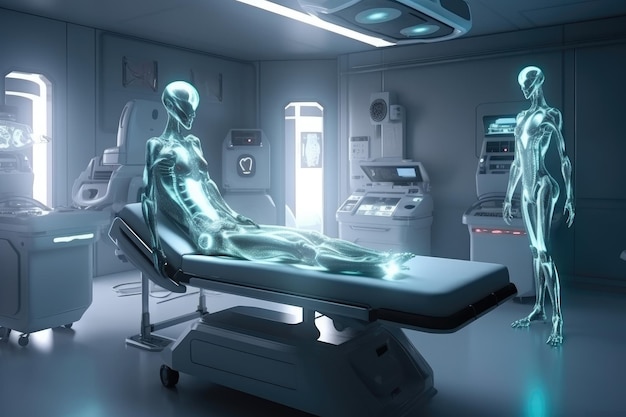This AI-generated digital illustration depicts a futuristic medical setting indoors, likely aboard a spaceship. The scene is dominated by two semi-transparent, bioluminescent alien female figures with glowing green skin, through which their rib structures and internal organs are visible. One alien is seated on a slightly inclined hospital examination bed positioned centrally in the room. She has an elongated face with a bulbous head and tapering chin, along with two breasts, hinting at a humanoid physiology. The other alien, featuring a similar anatomical structure, including a dome-like head and sharp chin, stands barefoot in the top right-hand corner in front of a gray medical equipment cabinet with a screen. The room itself is filled with futuristic medical equipment, overhead fluorescent lighting, and a console with a monitor. The lighting sources include ambient lights from the ceiling and illuminating a doorway in the background, as well as additional light from a window or entryway in the top left-hand corner. The color palette includes light blue, white, off-white, and black, enhancing the eerie, otherworldly atmosphere of the scene.